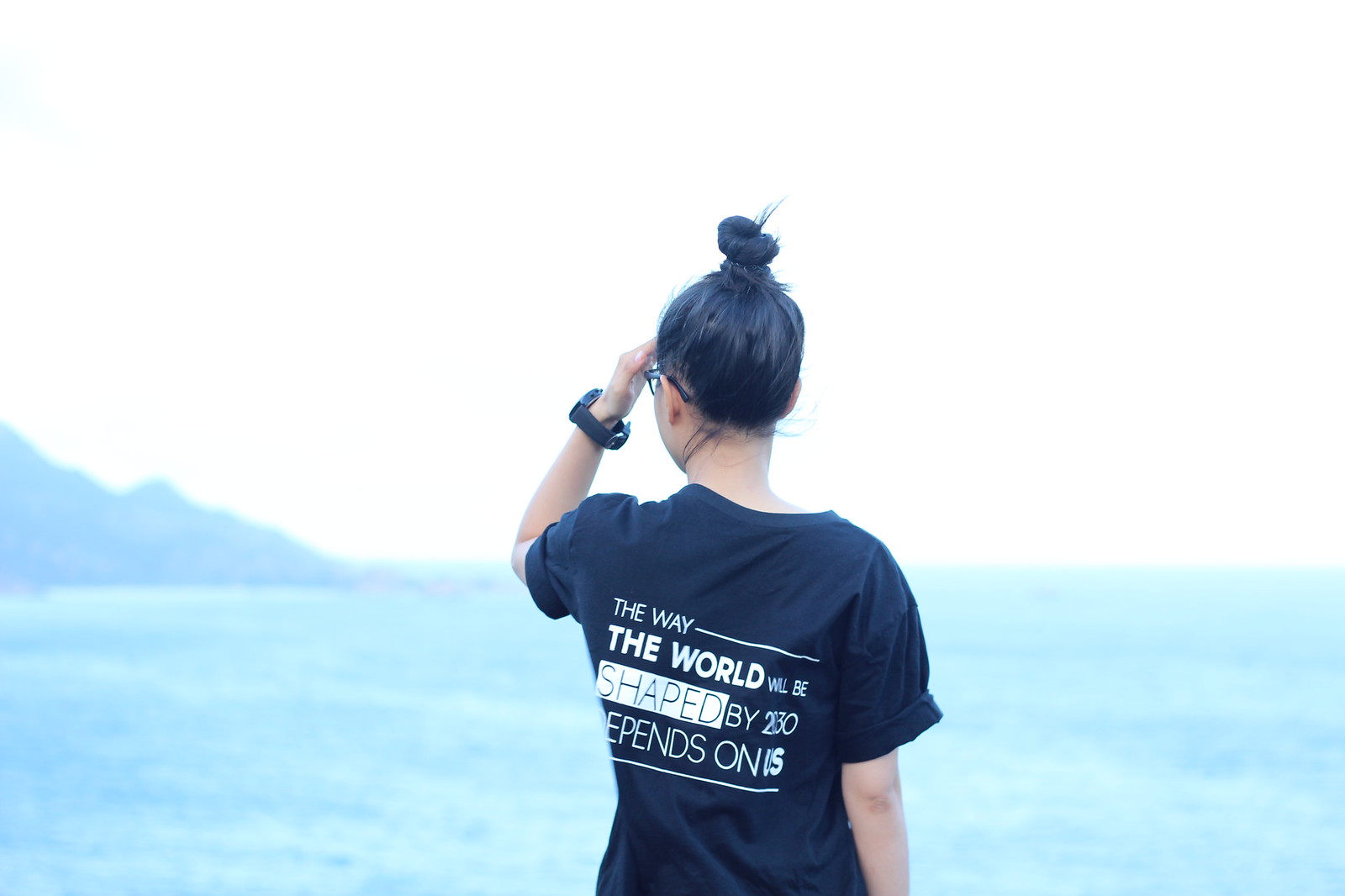The photograph, taken outside on a sunny day, captures the back of a girl as she gazes across a blue ocean. Her black hair is tied in a high bun, and she is wearing glasses and a black wristwatch on her left wrist. She raises her left hand to shield her eyes from the sun. She is dressed in a black t-shirt, the sleeves rolled up, with white text on the back that reads, "The way the world will be shaped by 2030 depends on us." The background is predominantly blue, with the ocean slightly out of focus, and a rocky outcropping of land visible on the left side under a bright, white sky.